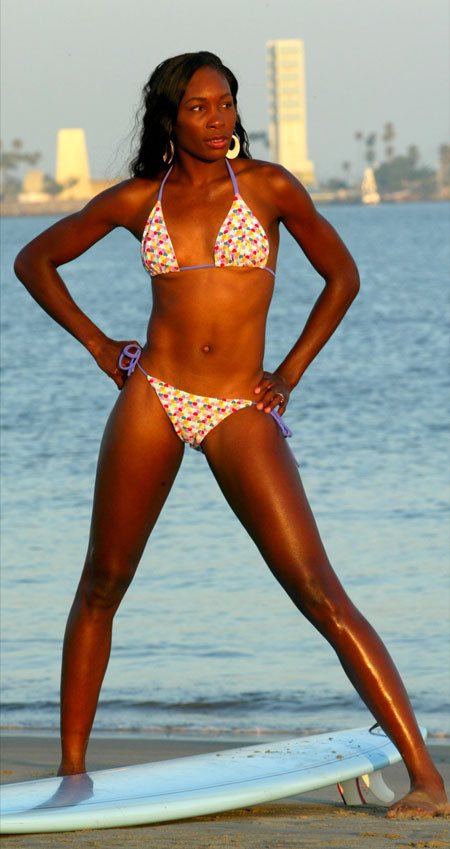This image features a tall, fit black woman standing confidently on a sandy beach, with calm ocean waters and a horizon lined with large white buildings and palm trees in the distance. She has long black hair and is wearing white hoop earrings. Her small bikini is predominantly white, adorned with a vibrant pattern of colorful circles in red, orange, green, purple, and yellow, and held together with light purple straps. She's striking a pose with legs spread and hands on her hips, standing over a white surfboard. The sky above is slightly blurry, suggesting an evening setting with an orange glow, hinting at sunset. Her gaze is directed to the side, not straight on, adding to the dynamic nature of the pose. There's a noticeable detail of sand on her feet, anchoring her in the beach environment.